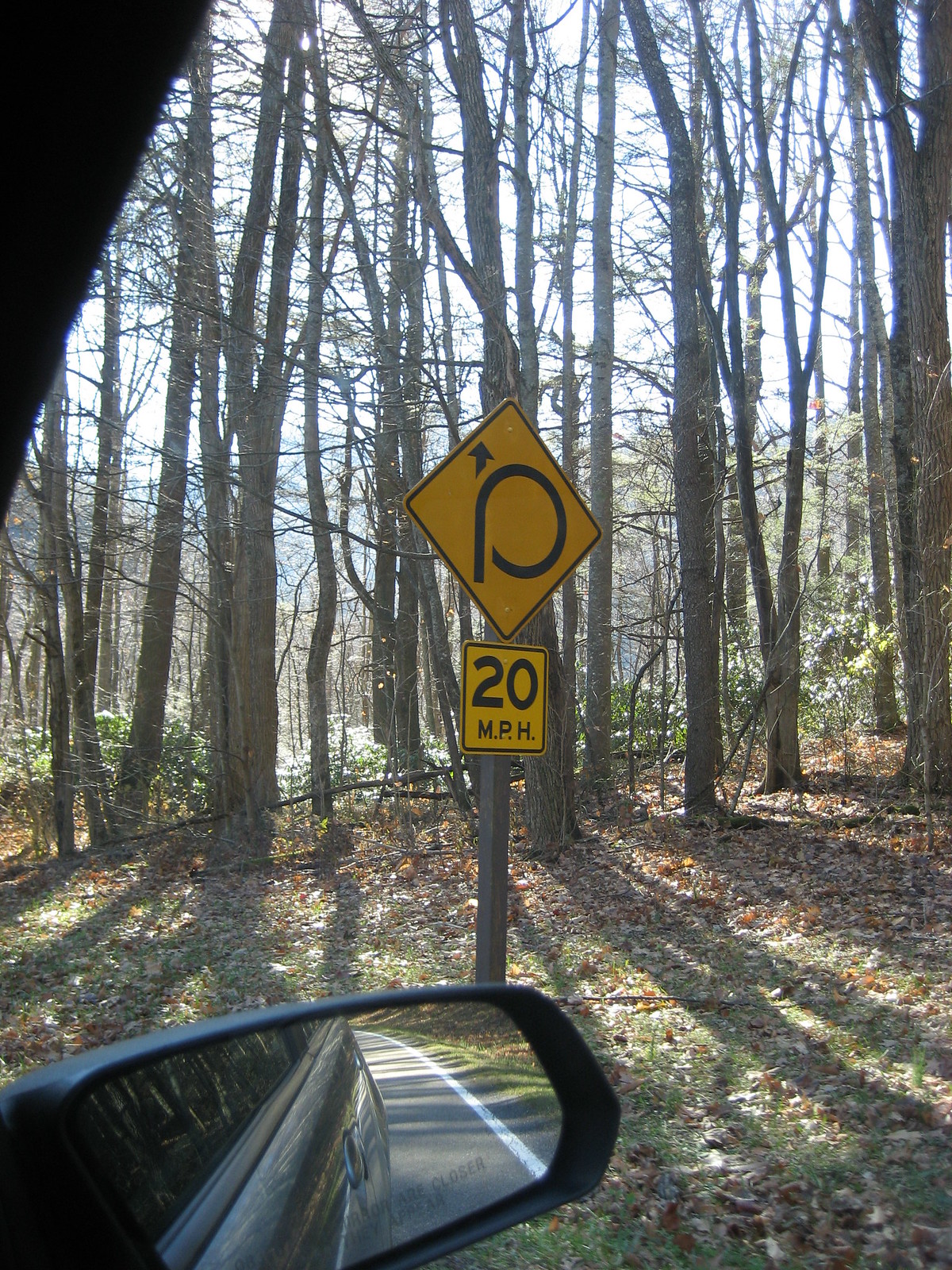In this image, we see a serene light woodland filled with tall, relatively young trees, their trunks slender and lofty as they stretch towards the sky. Sunlight filters through the dense greenery, illuminating patches of the forest floor and casting gentle shadows.

At the center of the image, a notable yellow diamond-shaped traffic sign stands out against the natural backdrop. This sign, tailored for motorists, features a bold 'P' with the head of an arrow pointing upward, and clearly indicates a speed limit of 20 miles per hour. The sign is affixed to a sturdy metallic post, securing its presence in the woodland.

In the foreground, the viewer's perspective is intriguingly anchored beside a tree and a car. The car's side mirror reflects a segment of its own body, which is juxtaposed against a glimpse of a roadway marked with a distinct white stripe. This composition hints at the proximity of civilization and nature, merging the quiet stillness of the woods with the subtle reminder of nearby vehicular activity.